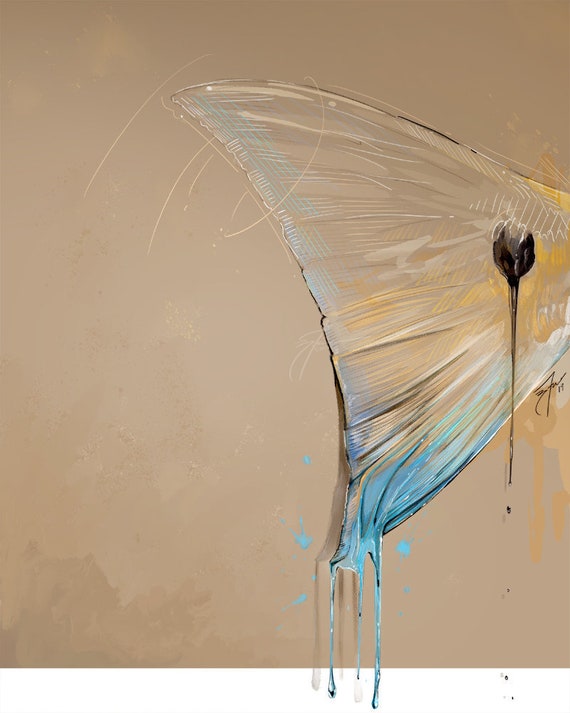The painting depicts a detailed and vibrant depiction of a translucent wing, resembling a hybrid between a dragonfly and a butterfly wing. The wing extends from the right side to the middle of the canvas and features intricate, white stripe patterns, lending it a glass-like, almost ethereal appearance. The background is predominantly a warm brown with darker spots, especially concentrated in the bottom left corner. 

At the bottom of the wing, a vivid blue substance appears to drip and pool, reminiscent of melting glass or blue blood, further accentuating the delicate nature of the wing. The colors in the painting include shades of blue, tan, black, orange, yellow, and gray. There is also a notable black spot on the wing. 

The painting captures a blend of realism and surrealism with the meticulous portrayal of the wing's translucency and the bold, dripping colors. Adding to the artistic composition, there is a signature located on the right side beneath the wing, indicating the artist's mark.